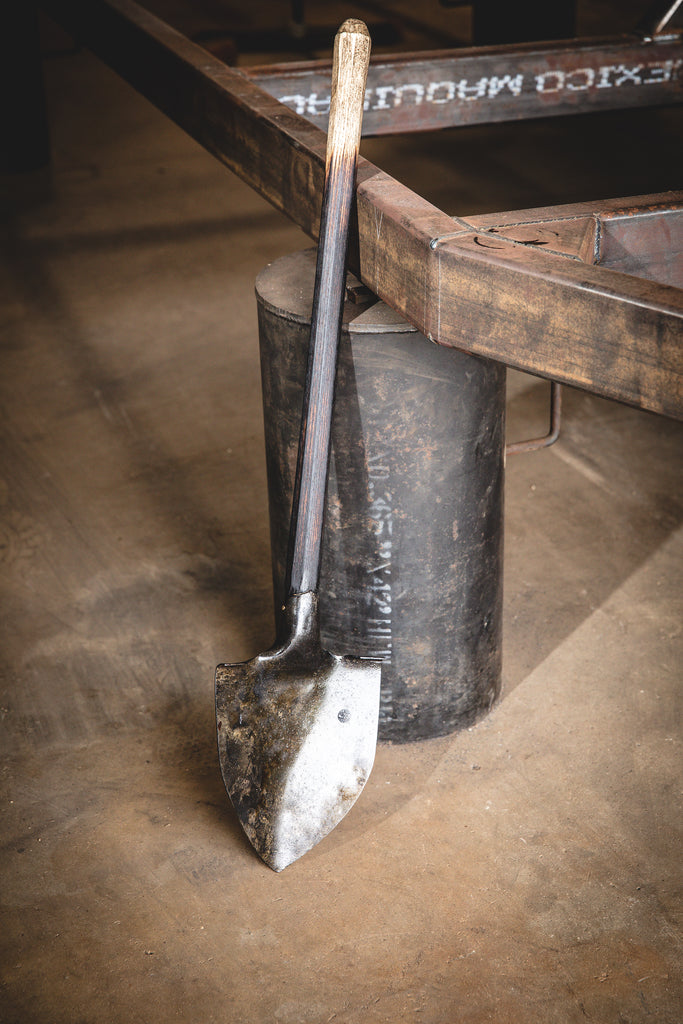In this photograph, a worn shovel leans against a dark, cylindrical metal post with a flat top. The shovel has a pointed, silver-to-dark colored blade and a wooden handle, with the lower part of the handle stained darker than the upper portion. The post, which supports a partially visible metal frame that resembles a small trailer or cart, has white numerical markings on its side, possibly including the numbers six, five, four, or two. The ground in the scene is a dirty, brown concrete floor, adding to the overall neglected and unclean appearance of the surroundings.